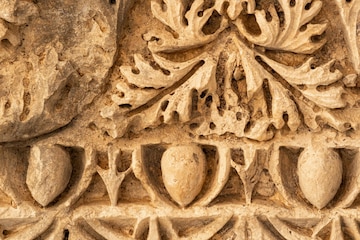The image appears to depict a horizontal rectangular section of a carved molding, likely made from wood, clay, or a similar material. The predominant color is a light tan or beige, mimicking natural wood tones. At the top left, there is a semicircular element resembling a carved rock. To the right of this, the main focus features intricately carved leaves, with three leaves facing down and three facing up to the left. Below the leaves, there is a small ledge or shelf supporting three almond-shaped carvings that resemble acorns. The design continues with additional carved patterns, although part of the lower section is cut off, making it difficult to discern the complete details. The craftsmanship is highly detailed, suggesting the image captures an ornate piece of decorative molding.